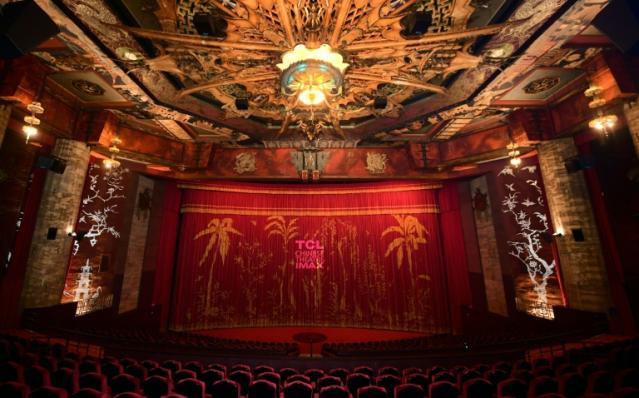The image captures a theater from a crowd perspective, centered on a large, ornate stage. The stage features a lush red curtain with gold borders and embroidered gold palm trees. In the center of the curtain, the letters "TCL" are visible in pink. The red floor compliments the rich aesthetic of the curtain. Flanking the stage on both sides are grand marble pillars with accents of red wood. The ceiling is adorned with a large chandelier, which has intricate designs resembling a flower with a central white and orange light, surrounded by greenish-blue and orange glass. Above the stage, the wall has red woodwork with elaborate embroidery. The chairs, visible from the bottom of the image, are padded and covered in red velvet, adding to the theater's opulent atmosphere. The ceiling also features detailed artwork extending along its sides, enhancing the theater's luxurious feel.